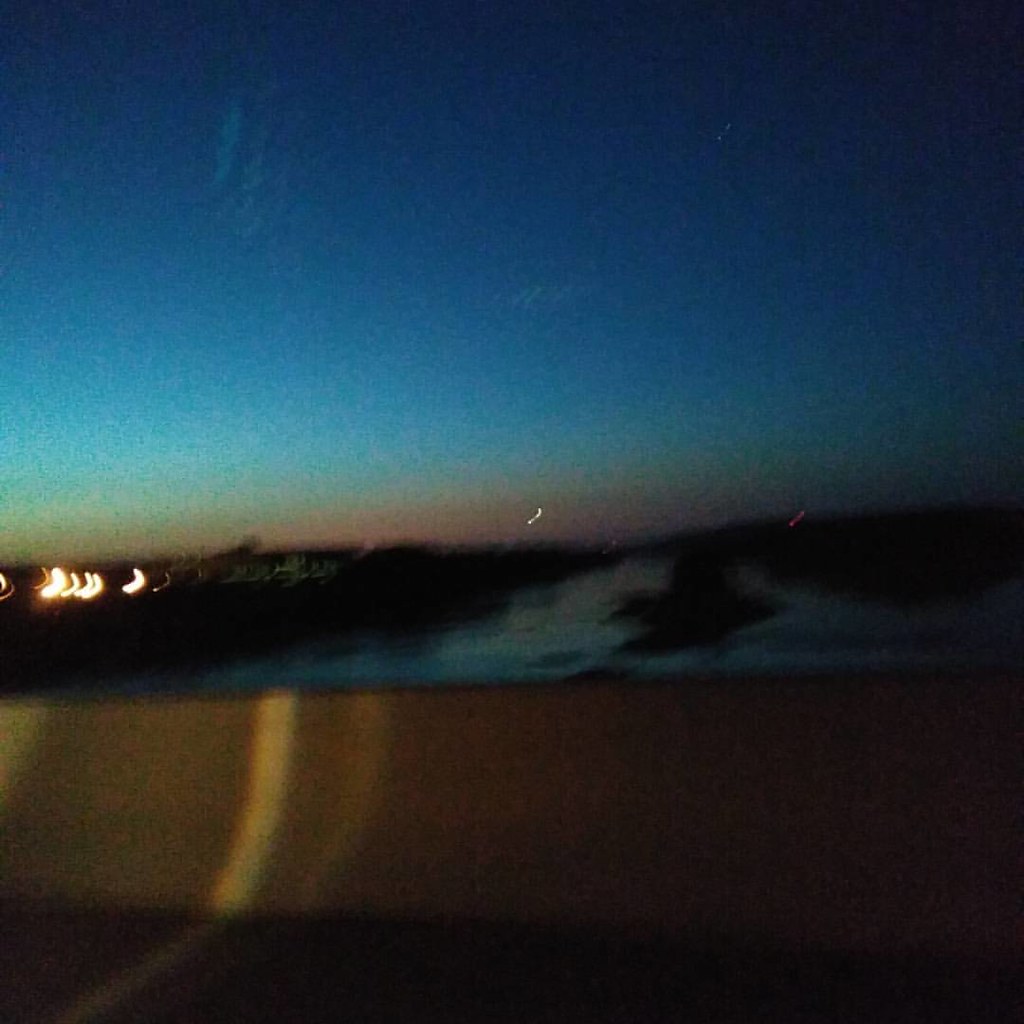A blurred, square photograph captures a scene through a passenger side window, revealing the reflective distortion of the glass. Taken at night or during dusk, the sky transitions from a deep blue at the top to a warm orange near the horizon, indicating the time of day. The lower portion of the image features a gold reflective surface, possibly the car panel or streetlights, while the middle left section shows multiple headlights from oncoming or adjacent vehicles. The combination of reflections and blurry elements evokes a sense of motion and transient beauty.